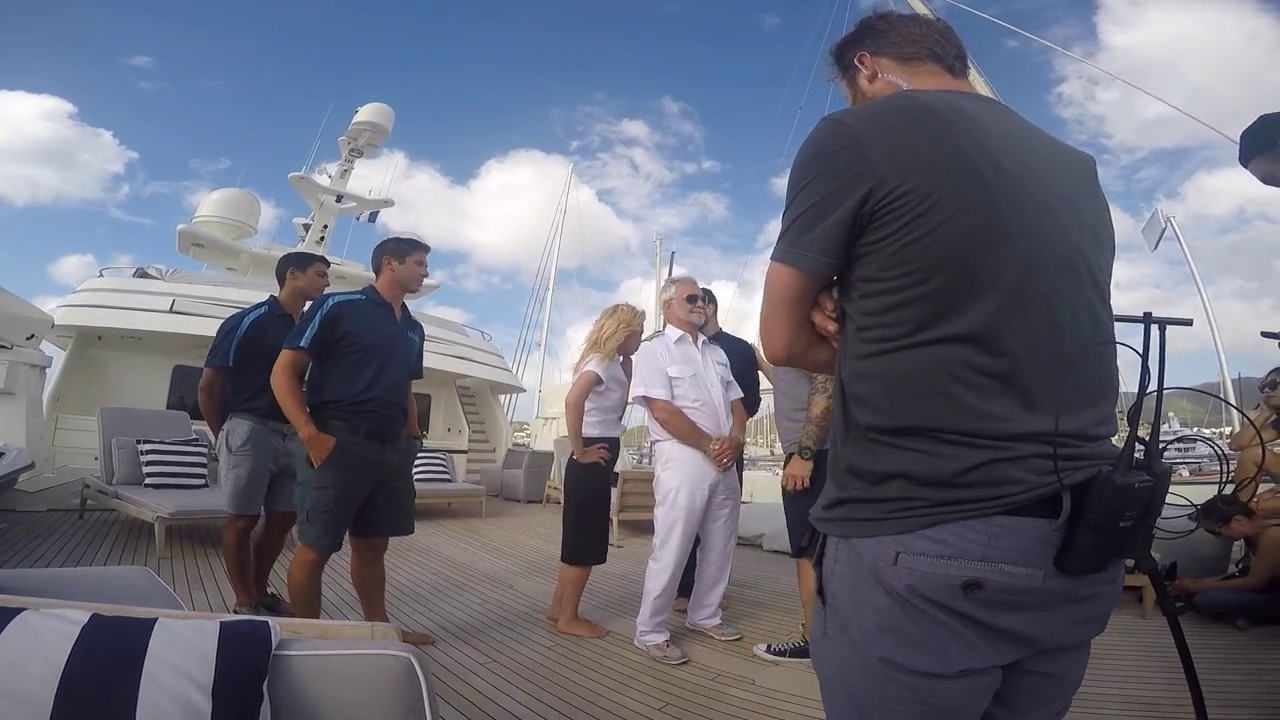The image captures a scene of a bustling marina, featuring a wooden planked deck teeming with activity, likely from the filming of a reality television show. In the background, a large cruiser or yacht is visible, enhancing the nautical ambiance. Central to the scene is a distinguished white-haired gentleman who appears to be the skipper, dressed entirely in white with a button-up shirt and sunglasses, hands clasped in front of him. Positioned around the captain are several individuals, all seemingly involved in the production or as part of the boat crew.

A blonde-haired woman, clad in a white shirt and black skirt with hands on her hips, stands behind the skipper. Next in line are two younger men dressed alike in blue polo shirts and shorts, with their hands in their pockets. The person in the foreground, possibly a production crew member, has their back to the camera and features a noticeable battery pack or mic pack extending from their back pocket. The detailed ensemble reveals a vibrant mix of relaxation and structured activity, all under the warm embrace of a sunny day, with everyone dressed appropriately for the warm weather.